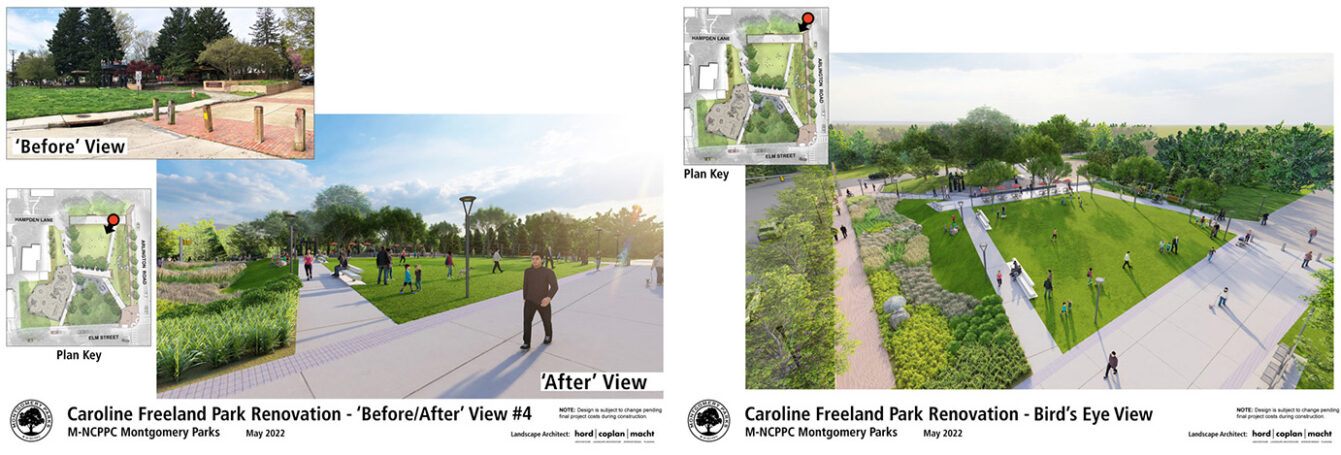This image comprises two detailed diagrams depicting the renovation plans for Caroline Freeland Park. On the left side, titled "Caroline Freeland Park Renovation before/after view number four," a composite image captures the park's transformation. The 'before' view showcases a plain green grassy field with a brick path and bollards, flanked by trees in the background. The 'after' view illustrates the same space post-renovation, now featuring a concrete path, landscaped gardens, and an active scene with numerous people and children engaging in activities under a bright blue sky.

On the right side, the image is labeled "Caroline Freeland Park Renovation bird's-eye view." This overhead depiction includes a plan key in the upper left corner illustrating the layout and pathways of the park. The bottom portion offers a realistic visualization of the renovated park, showing the newly added concrete path, the grassy field, the placement of trees, and additional landscaping features. Both diagrams provide comprehensive visual details from different angles, highlighting the extensive changes implemented in the renovation project.